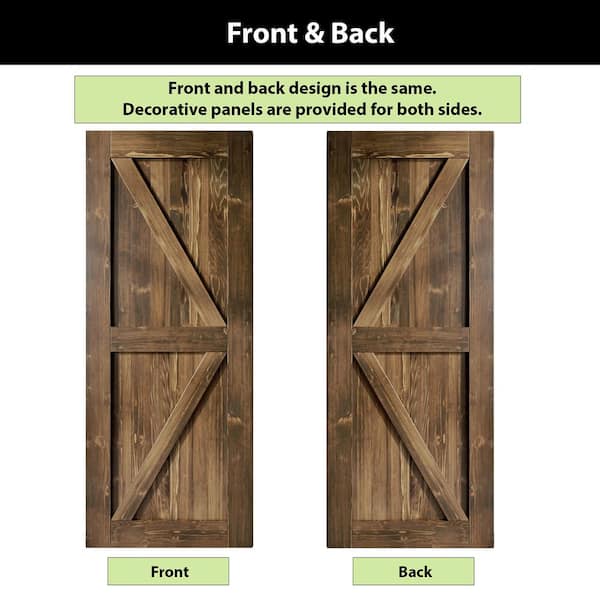This infographic showcases options for purchasing wooden planked sliding barn doors. It features two photographs of the doors side by side. At the top, a black text bar labeled "Front and Back" identifies the images. Beneath it, a green text bar states, "Front and back design is the same. Decorative panels are provided for both sides." The first photograph displays the front view of a wooden planked sliding barn door, with a label below reading "Front." The second photograph shows the back view of the same door, similarly labeled "Back." This comprehensive layout ensures that potential buyers can see both sides of the doors, fully illustrating their uniform design.